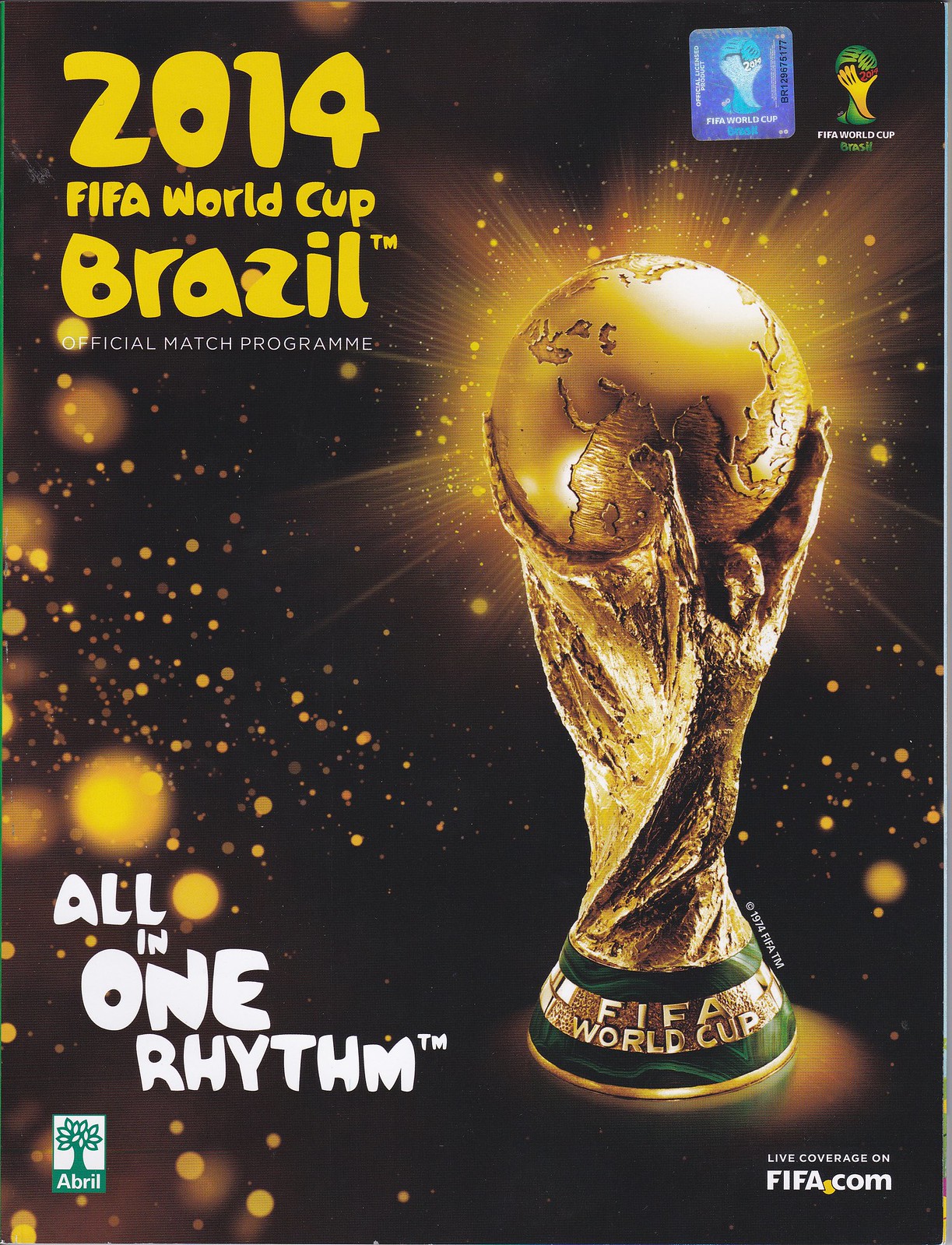This is the front cover of the official match program for the 2014 FIFA World Cup in Brazil. The cover features a vertical rectangular design with a predominantly black or deep brown background. At the center-right, there is a golden globe held by a statue that resembles hands or claws embracing the world. The globe emits yellow-orange light bursts and sparkling stars that extend across the cover. The base of the statue is green with gold accents, inscribed with "FIFA World Cup."

In the upper left-hand corner, "2014 FIFA World Cup Brazil" is written in yellow-gold font, accompanied by "Official Match Program" underneath in white. The lower left-hand corner displays the phrase "All in One Rhythm" angled diagonally over four lines. Below this, there is a white square with a green tree logo representing the sponsor, Abril. The lower right-hand corner includes the text "Live Coverage on FIFA.com," with "fifa.com" more prominently displayed. The top right-hand corner features a blue square with the FIFA World Cup logo, and next to it, a green and gold image with "2014" written in red above "FIFA World Cup Brazil."